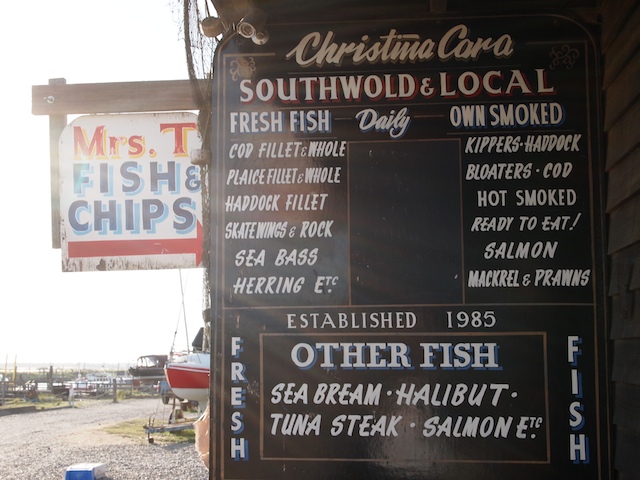This photograph features the detailed signage of a fish and chips store. To the left, a smaller sign reads "Mrs. T Fish and Chips" in red and blue font with a red arrow pointing right. The larger, prominent black sign on the right is headed with "Christina Cara", followed by "South, Wooled, and Local", which announces the establishment's specialty in fresh and smoked fish. 

The left column lists fresh fish options such as Cod Fillet, Plaice Fillet and Whole, Haddock Fillet, Skate Wings, Rock, Sea Bass, and Herring. The right column details the smoked fish selections including Kippers, Haddock, Bloaters, Cod, Hot Smoked Ready to Eat, Salmon, Mackerel, and Prawns. The bottom half of the sign, labeled "Established 1985", offers additional fresh fish like Sea Bream, Halibut, Tuna Steak, and Salmon. The sign's black backdrop with white text contrasts effectively, ensuring clear readability.

The setting is outdoors, with subtle hints of a serene lake and the bow of a boat visible in the background, enhancing the rustic, nautical ambiance of the scene.